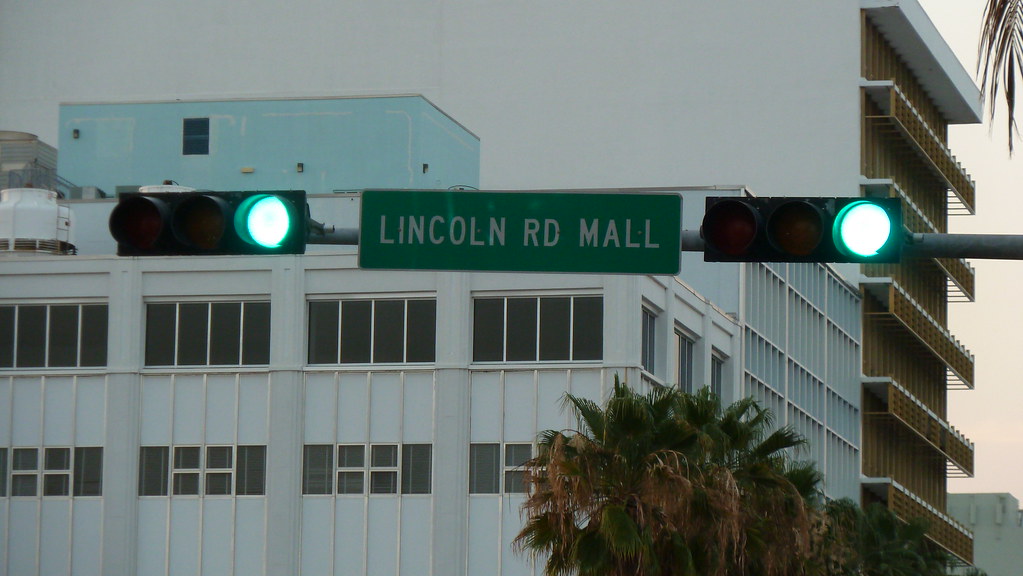The photograph depicts a zoomed-in view of a horizontally-oriented traffic light, where all three lights are lined up horizontally instead of vertically. There are two active green lights flanking a green road sign that reads "Lincoln Road Mall" in white text. This setup is affixed to a gray or black pole positioned over a roadway intersection.

The scene appears to be shot looking upwards, as if from the perspective of someone sitting inside a car, peering through the windshield. Surrounding the traffic light, the backdrop contains a variety of buildings and foliage, emphasizing the location's urban yet green environment. A prominent white building is visible, showcasing several rows of windows. A smaller, mint-green structure with a single window and some vents is perched on top of this white building.

Adding to the tropical ambiance, several palm trees with green and some brown fronds stand near the buildings, suggesting a warm climate, possibly hinting at a location like California. Additional buildings are present in the background: a brown building with white trims and a light gray building, completing the layered urban scenery visible in this high-angle photograph.